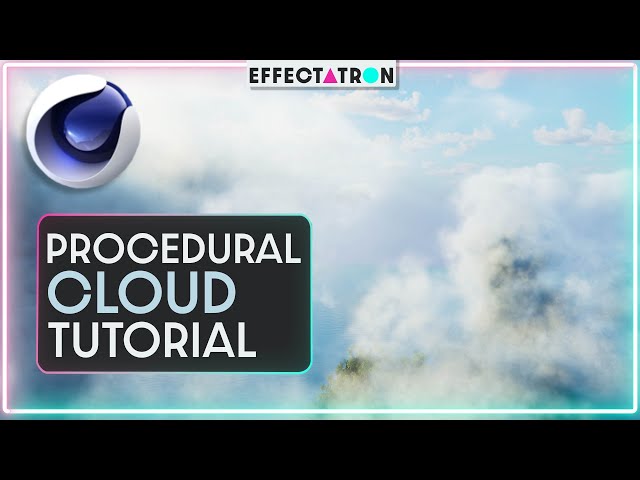The image primarily showcases a computer monitor bordered on the top and bottom by thick black bars. At the very top center of the screen, under the top black section, it prominently displays the text "Effectatron" where the 'A' is stylized as a purple triangle and the 'O' as a light blue circle. The monitor's background reveals a vibrant blue sky filled with large, puffy, white clouds, some darker and more painted in appearance, creating a dynamic skyscape.

In the top left corner of the screen, there's an abstract, futuristic object resembling a round, white camera with a blue, reflective center. Below this object, situated in the bottom left corner of the monitor, there's a dark gray rectangular box with a white outline. This box contains bold white text that reads "Procedural Cloud Tutorial," emphasizing "cloud" in light blue. The entire scene gives the impression of an advertisement or tutorial for generating procedural clouds, visually immersing the viewer as if flying through the clouds.